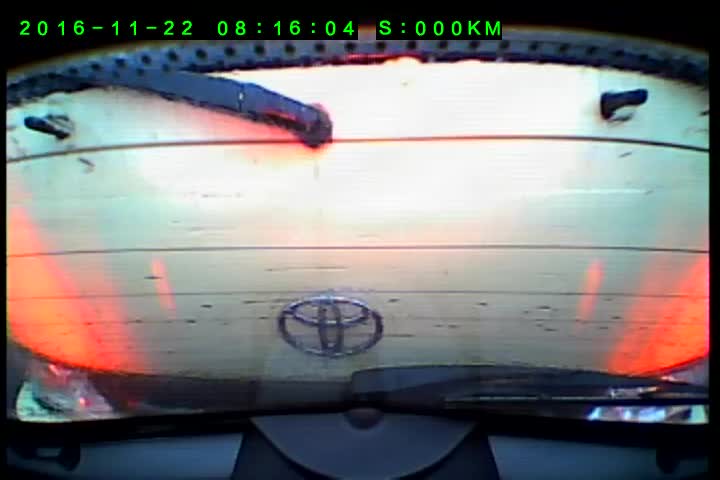The image is a detailed screen capture displayed on a monitor or TV, showcasing a scene inside a Toyota vehicle. At the top of the screen, in bright green and computer-like text, is the timestamp "2016-11-22 08:16:04 S:000KM." The view is from within the cargo area, directed outward, possibly towards a garage door. The upper part of the image contains a windshield wiper, horizontal white lines resembling boards, and a distinctive silver Toyota logo prominently displayed. Below the logo is a dark black plastic base, which supports the monitor. To the left, there is an elongated black strip, peppered with small holes. The foreground suggests a white vehicle with elements such as handles and emblem details that hint at its make, though the overall scene remains anchored by the identifiable Toyota logo.